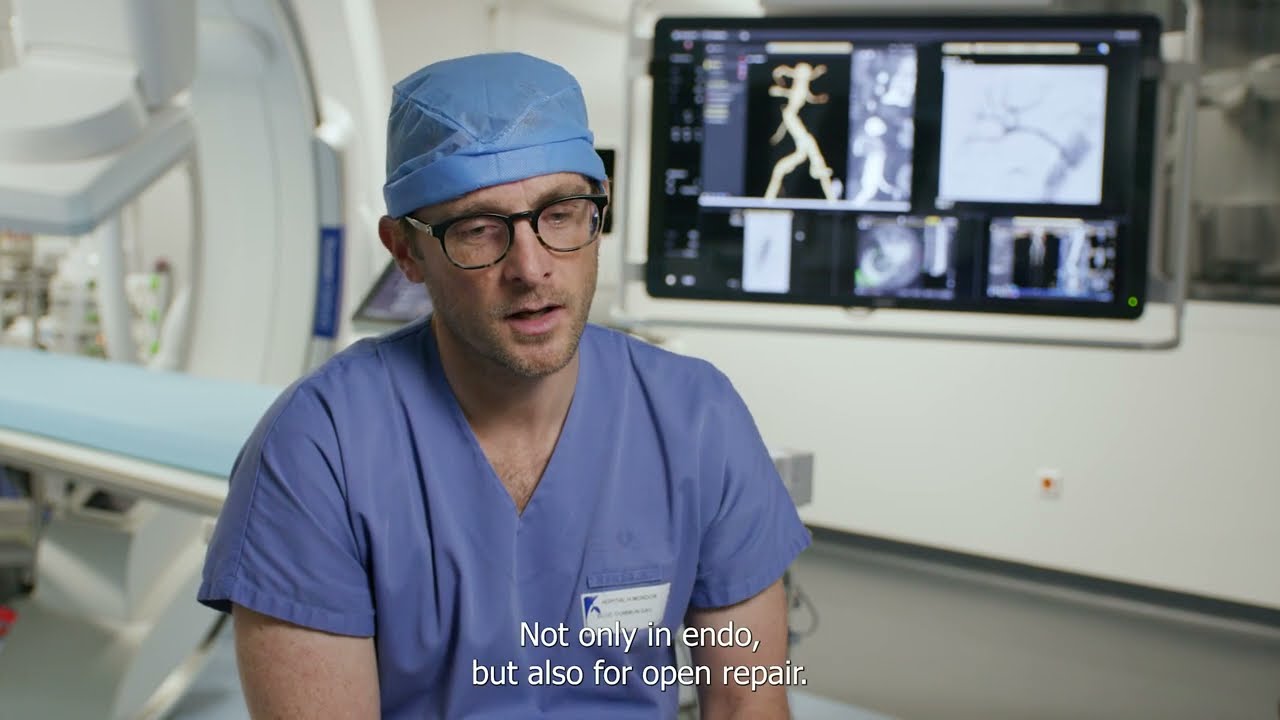In the center of the image stands a middle-aged male doctor wearing light blue scrubs and a matching blue cap. He sports black-framed glasses and has a white name tag on his left chest. The scrubs feature a V-shaped collar and short sleeves. Behind him to the left is a circular MRI machine, accompanied by a long bed with a light blue mattress on top. To the right, mounted above a white wall, is a large digital screen displaying various images of human body parts and cells. The scene is set against a gray floor. In white text at the bottom of the image, it reads: "Not only in ENDO, but also for open repair."